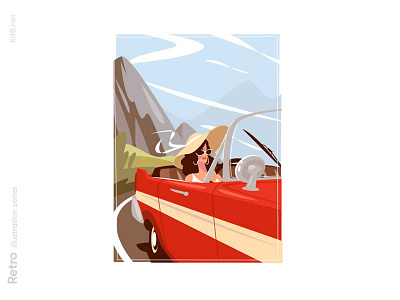This small, vertically aligned, computer-generated image portrays a young woman seated in the front passenger seat of a classic red convertible, adorned with a white horizontal stripe down its side. The car, which also features a windshield, windshield wipers, a side mirror, door handle, and back bumper, is depicted driving along a mountain road with brown and tan peaks in the background under a light blue sky filled with white, swirling clouds.

The woman, with curly, wavy brown hair, dons a wide straw sun hat with a white ribbon blowing in the wind, complementing her white sunglasses, white top, and elegant white earrings. Her red lipstick adds a touch of glamour to her retro look. Although only the right side of the car and the back right wheel are visible, the entire scene is part of a "Retro Illustration Series," as indicated by the vertical text against a white background.